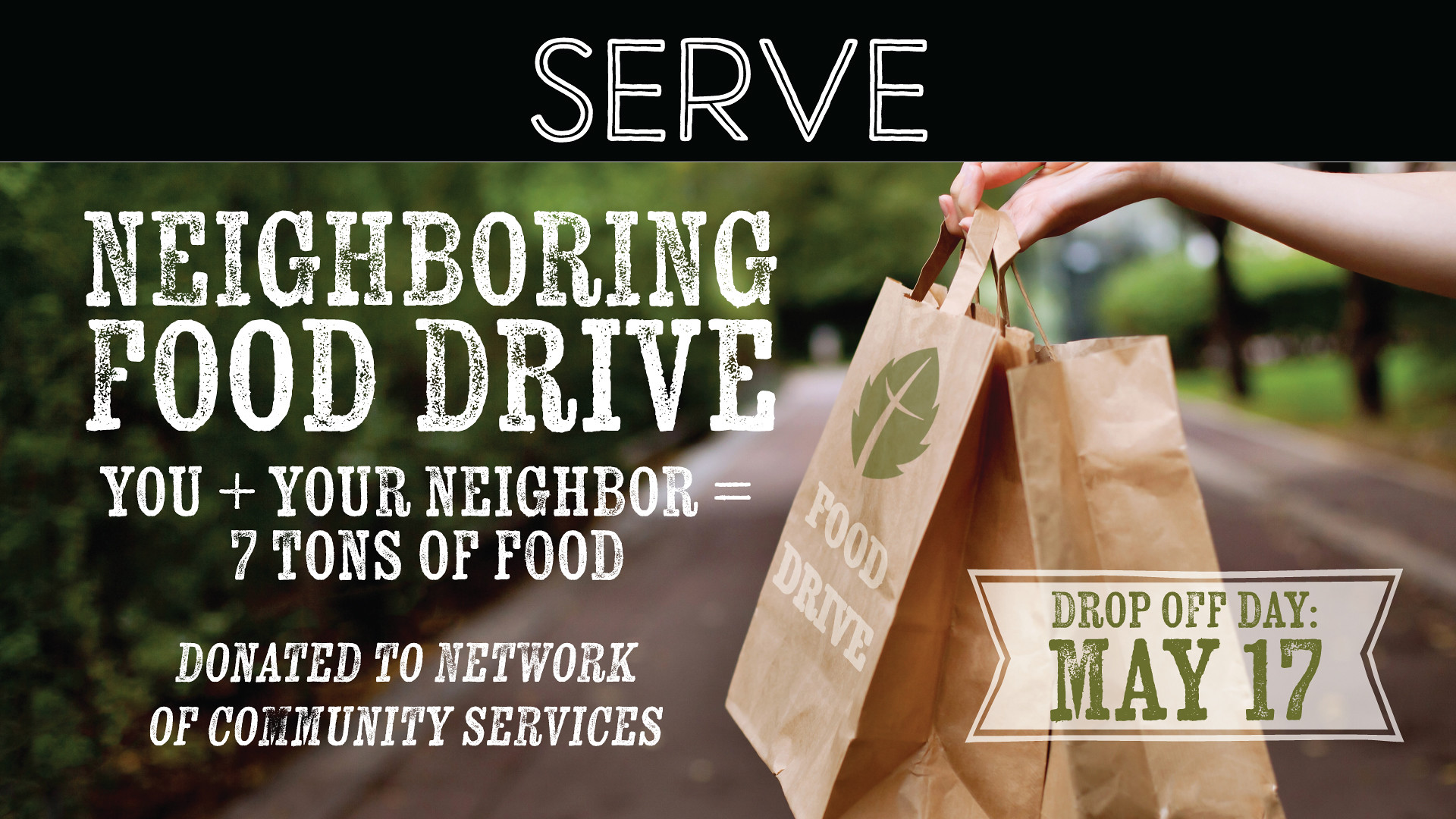This wide rectangular image features an advertisement centered around a community food drive. Dominating the top portion, a thick black bar runs horizontally across the image with the word "SERVE" boldly inscribed in white capital letters. Below this bar, the background consists of a blurry road that extends and converges into the horizon at the center, flanked by green trees on the left and a grassy area on the right. 

Emerging from the top right side is a white hand holding two light brown paper grocery bags, each adorned with a green leaf and the text "FOOD DRIVE." Additionally, a green banner on one of the bags indicates "Drop-off Day, May 17th" in white text. 

To the left of the image, written in white font, are the words: "NEIGHBORING FOOD DRIVE. YOU + YOUR NEIGHBOR = 7 TONS OF FOOD DONATED TO NETWORK OF COMMUNITY SERVICES." This text highlights the collaborative effort and impact of the community food drive, all set against the blurred backdrop of a serene road and vibrant greenery.